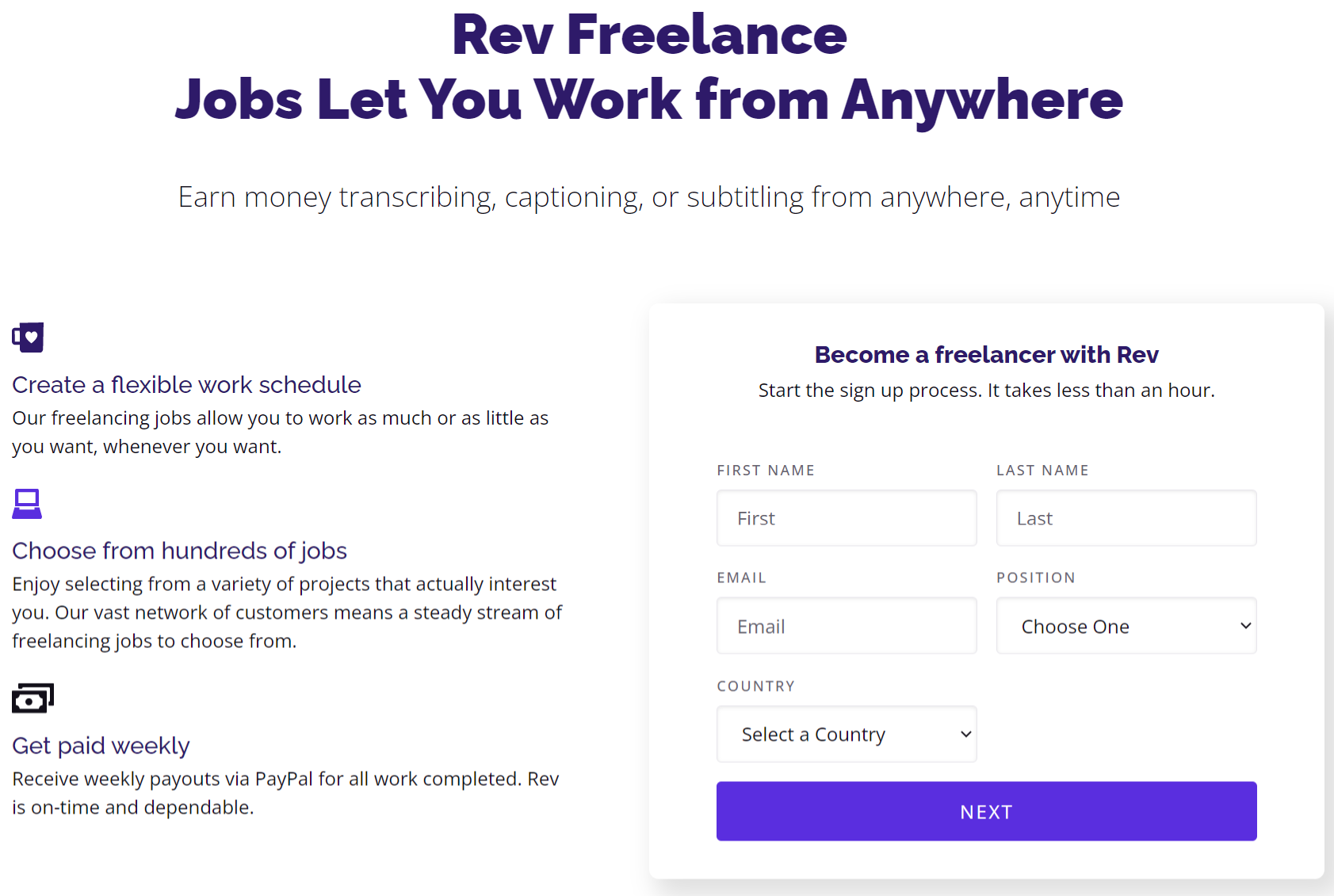The image showcases the homepage of a website called "Rev Freelance." At the top of the page, there's a prominent banner with the text "Rev Freelance" in bold purple letters, followed by the slogan "Jobs let you work from anywhere." Beneath the banner, a smaller, finer black font adds more detail, stating, "Earn money transcribing, captioning, or subtitling from anywhere, anytime."

On the left-hand side of the page, several benefits of joining Rev Freelance are highlighted:
1. **Create a Flexible Work Schedule:** The freelancing jobs at Rev allow users to work as much or as little as they desire, whenever they wish.
2. **Choose from Hundreds of Jobs:** Freelancers can select from a wide variety of projects tailored to their interests.
3. **Get Paid Weekly:** Rev ensures timely and dependable weekly payouts via PayPal for all completed work.

To the right of these details, a panel invites users to become freelancers with Rev. The sign-up process includes fields for a first name, last name, email address, the desired position, and the country of residence. A purple "Next" button at the bottom of the panel enables users to move forward to the next step of the registration process.